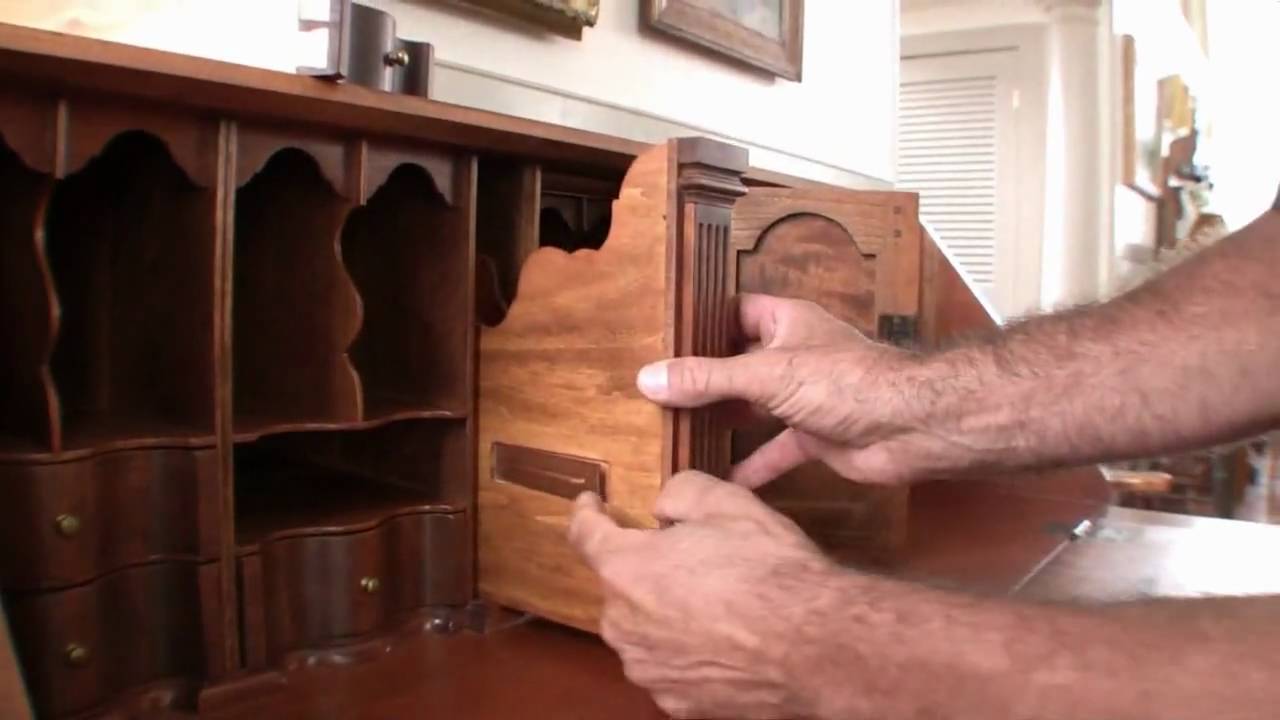The image shows an early 19th-century hardwood secretary desk, likely made from oak, placed against a white wall. The desk features multiple slots and hidden compartments for various storage purposes. A man's hands are visible in the image, demonstrating how a customized wooden file holder or casing fits snugly into one of the slots. The desk's drawers and compartments, some with gold handles, appear to be crafted from different types of wood. In the background, there are several pictures with brown and gold frames, and a white cabinet door, adding further detail to the scene. The overall setup showcases the intricate design and functionality of the antique desk.